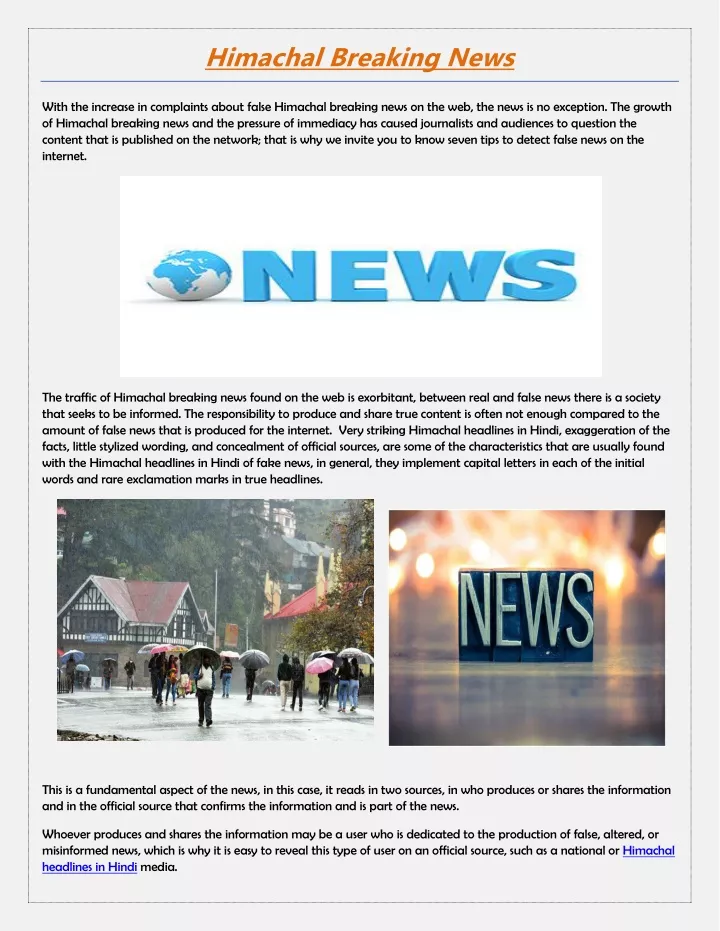**Hemishal Breaking News: Navigating the Storm of Misinformation**

In a captivating layout, Hemishal Breaking News presents a scene from a rainy day in a residential area. The central photograph captures individuals walking under umbrellas, epitomizing the daily hustle amidst downpour. To the right of this image, the latest news articles are featured, providing up-to-date information. 

Above this section, a striking banner displays the word "NEWS" in sky blue, alongside a stylized globe. The continents on the globe share the same sky blue hue, while the waterways are depicted in white, creating a modern and clean aesthetic.

The accompanying text highlights a pressing issue: the surge in complaints about false news circulating on the web, including Hemishal Breaking News. This phenomenon is linked to the relentless pressure for immediacy in news reporting, prompting both journalists and audiences to critically evaluate the published content.

The network addresses this concern by offering seven essential tips to detect false news online. They emphasize that the traffic for Hemishal Breaking News, encompassing both real and fake stories, is exorbitantly high. This reflects a wider societal hunger for information, which unfortunately leads to a proliferation of misleading content.

A particularly noticeable Hemishal headline in Hindi captures attention with its exaggerated facts, stylized wording, and lack of official sources. The use of capital letters for each initial word and rare punctuation, such as exclamation marks, often differentiates these fake headlines from genuine ones.

In the concluding section, the fundamental aspect of news integrity is underscored: the verification of information through reliable sources. The text cautions that individuals who produce or share false news are often detectable through official sources such as national Hemishal media in Hindi. These vigilant practices are essential for maintaining the credibility of the information consumed and shared in today's digital age.